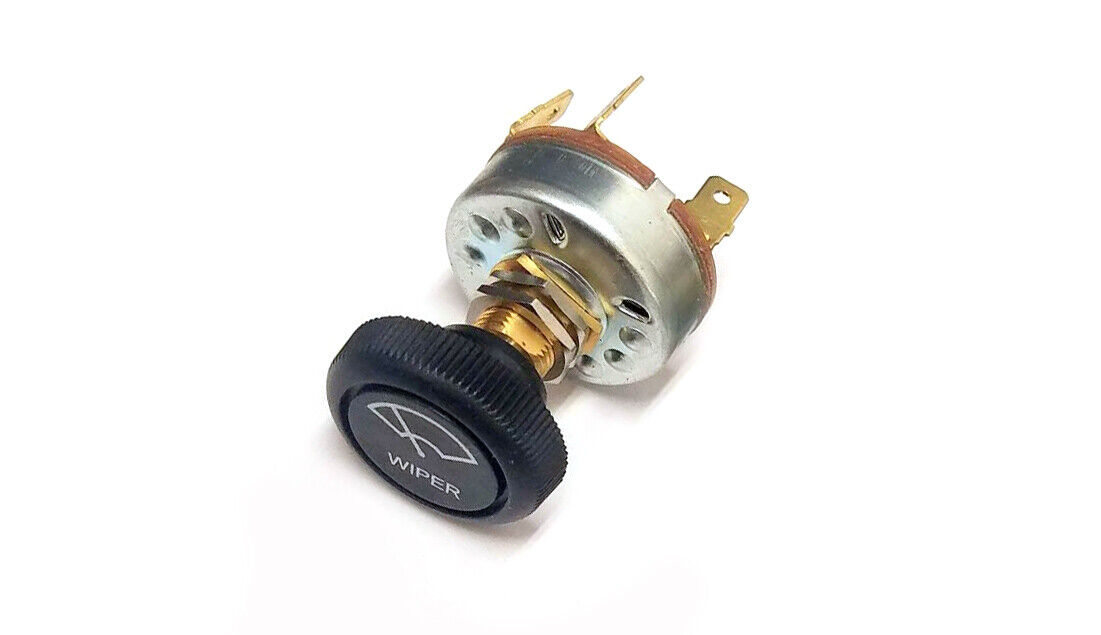The image depicts a detailed close-up of a car's windshield wiper control knob against a stark white background. The black, circular knob features a textured, grooved outer edge and prominently displays the word "WIPER" along with a white wiper symbol on its front face. This knob is oriented toward the bottom left corner of the frame. Connected to it is a brass fitting, which includes several washers and nuts. The brass fitting then attaches to a slender, cylindrical silver base, which appears to be inverted, with multiple screw holes visible. At the bottom of this cylindrical base, at least three brass-colored electrical plugs can be seen, suggesting that this component is designed to be wired into a vehicle's electrical system. The overall composition is highly realistic, emphasizing the mechanical details of the wiper control mechanism.